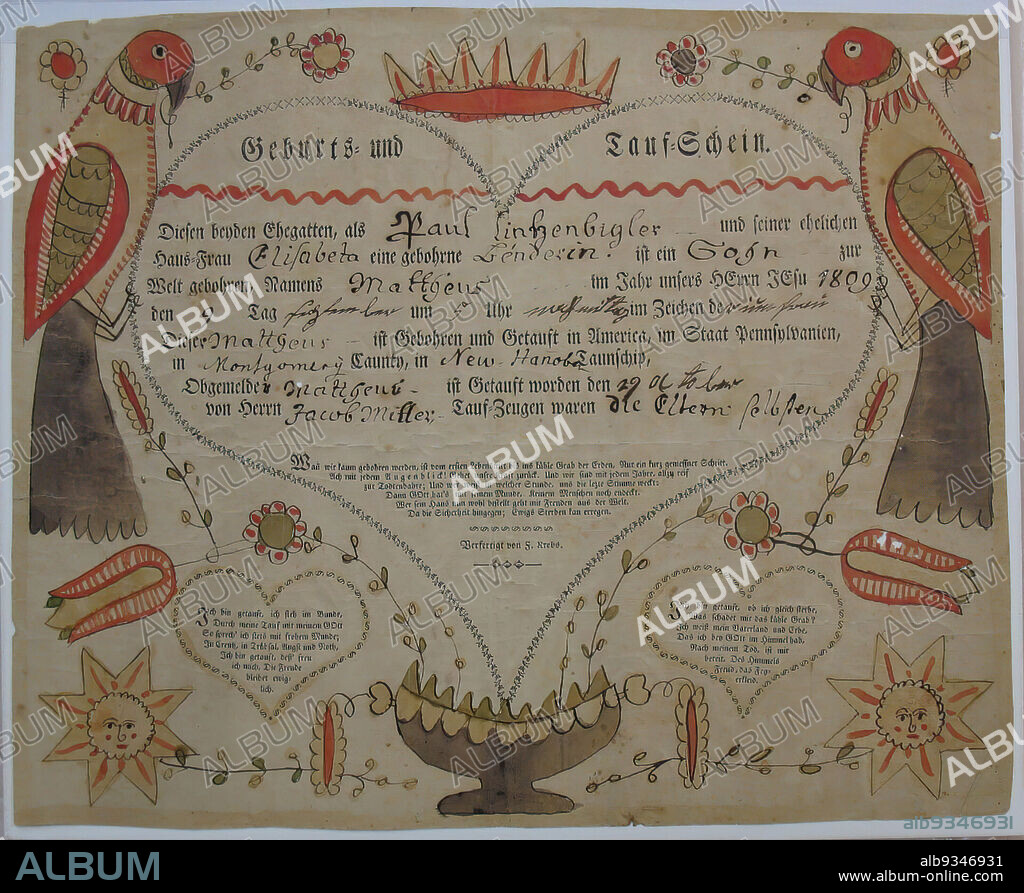This image appears to be a photograph of an old, intricately illustrated document, possibly a Pennsylvania Dutch or German marriage certificate. The paper has taken on a tea-stained tan and beige hue, indicative of its age. Dominating the center is a large heart filled with various signatures and foreign writing, likely in German. Flanking the heart, in the top corners, are two parrots adorned in a mix of orange, brown, olive, and yellow hues, holding orange flowers in their beaks. The parrots exhibit distinctive red heads, striped necks, brownish-red feathers, and blue tails. 

The illustration includes an array of decorative elements: a yellow and red crown at the top, suns with faces in the bottom corners, and numerous small hearts, flowers, and even a dish at the bottom with spikes reaching up towards the central heart. This entire page is overlaid with a watermark that repeatedly displays the word "album," and the bottom edge bears the URL "www.album-online.com." The combination of these elements, along with the heart motif, suggests the document is commemorating a wedding.